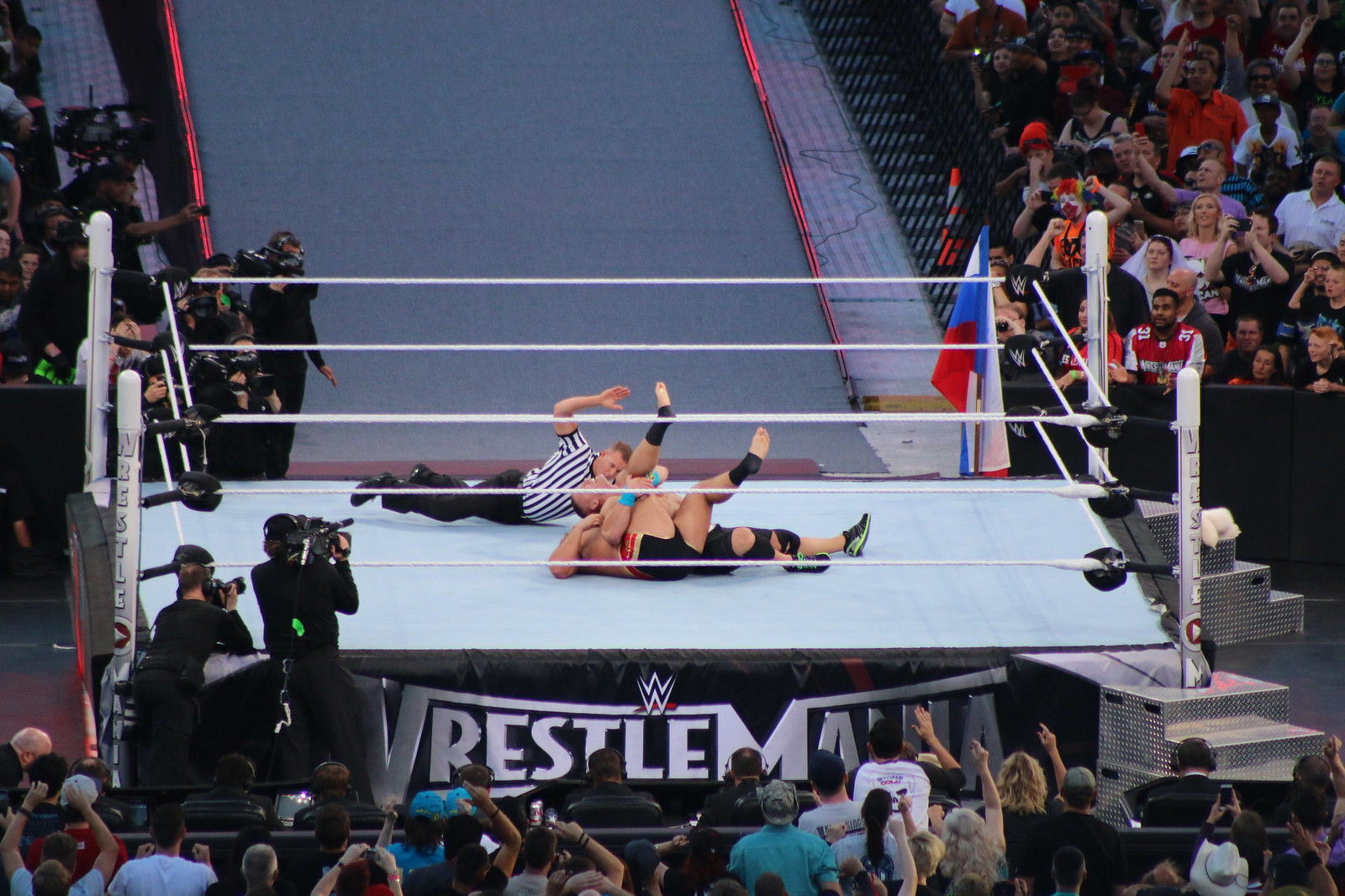This is a detailed color photograph of a WrestleMania event taking place inside a large stadium. At the center is a wrestling ring surrounded by white ropes, with the "WrestleMania" logo prominently displayed on the side. The action captures a crucial moment in the match: one wrestler has the other pinned by the leg while the referee, dressed in a black and white striped shirt, is poised on his front side to slap his hand on the ground, signaling the potential victory. Surrounding the ring are large groups of animated audience members, many of whom are wearing hats and shirts to show their support for their favorite wrestlers. In the foreground, cameramen are seen close to the ring, capturing the intense moment from different angles. The audience is visible on all sides, with hands raised and faces filled with excitement. Behind the ring, a large gray ramp extends out of sight, providing a grand walkway leading to the stage. A spacious path between two sections of the audience highlights the scale of the stadium and the magnitude of the event.